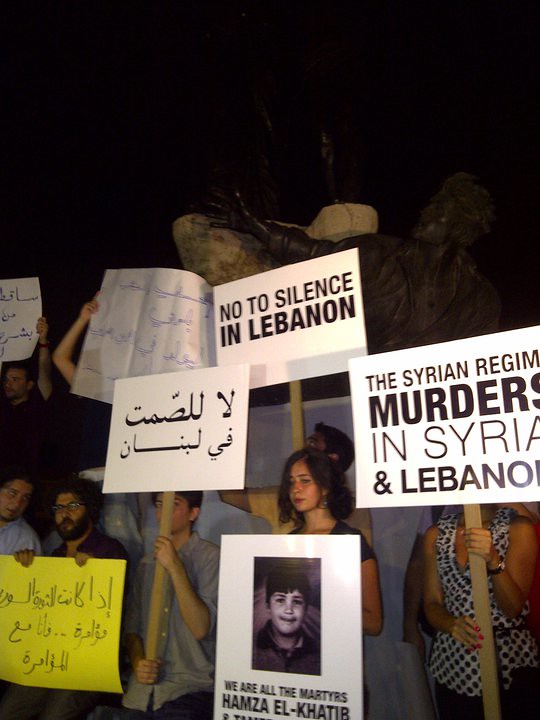The full-color nighttime photograph captures an intense outdoor protest featuring several younger individuals holding various protest signs. Both English and Arabic text are visible on the signs, reflecting the diverse messages of the participants. Central to the scene is a man holding a large yellow sign written in Arabic. Prominently, a woman displays a sign with the picture of a young boy and the caption, "We are all the martyrs, Hamza al-Khatib," commemorating the likely deceased boy. Another woman holds a sign that reads, "The Syrian regime murders in Syria and Lebanon," while another protester bears a sign stating, "No to silence in Lebanon." The atmosphere is charged with activism, underscored by the multilingual and graphic nature of the signs.